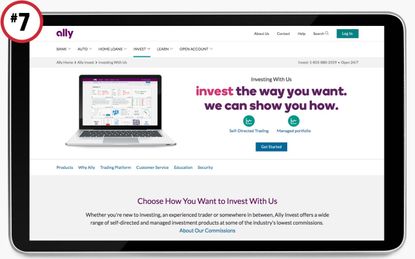The image is a small, left-to-right horizontal advertisement for Ally, showing a light gray border surrounding a tablet or iPad. The device displays a webpage with the Ally logo in purple at the top. The upper left-hand corner features a red circle with a white interior and a black number 7 in the middle. The webpage has a white background and a black border around the iPad.

Below the Ally logo, various black subheadings are available for clicking, with one highlighted by an underlined teal-green line. On the top right, the webpage includes navigation options such as About Us, Contact Us, Help, Search, and a green Login button within a rectangle with white text.

To the left of the iPad screen is an image of a laptop, showing some content. To the right of the laptop image, the text reads: "Invest. Increasing Investing with us. Invest the way you want. We can show you how." Various clickable icons in teal and blue are displayed below this section, offering different options related to their products and services.

At the bottom of the image, a black text caption reads: "Choose how you want to invest with us," accompanied by a blue clickable link about their commissions.